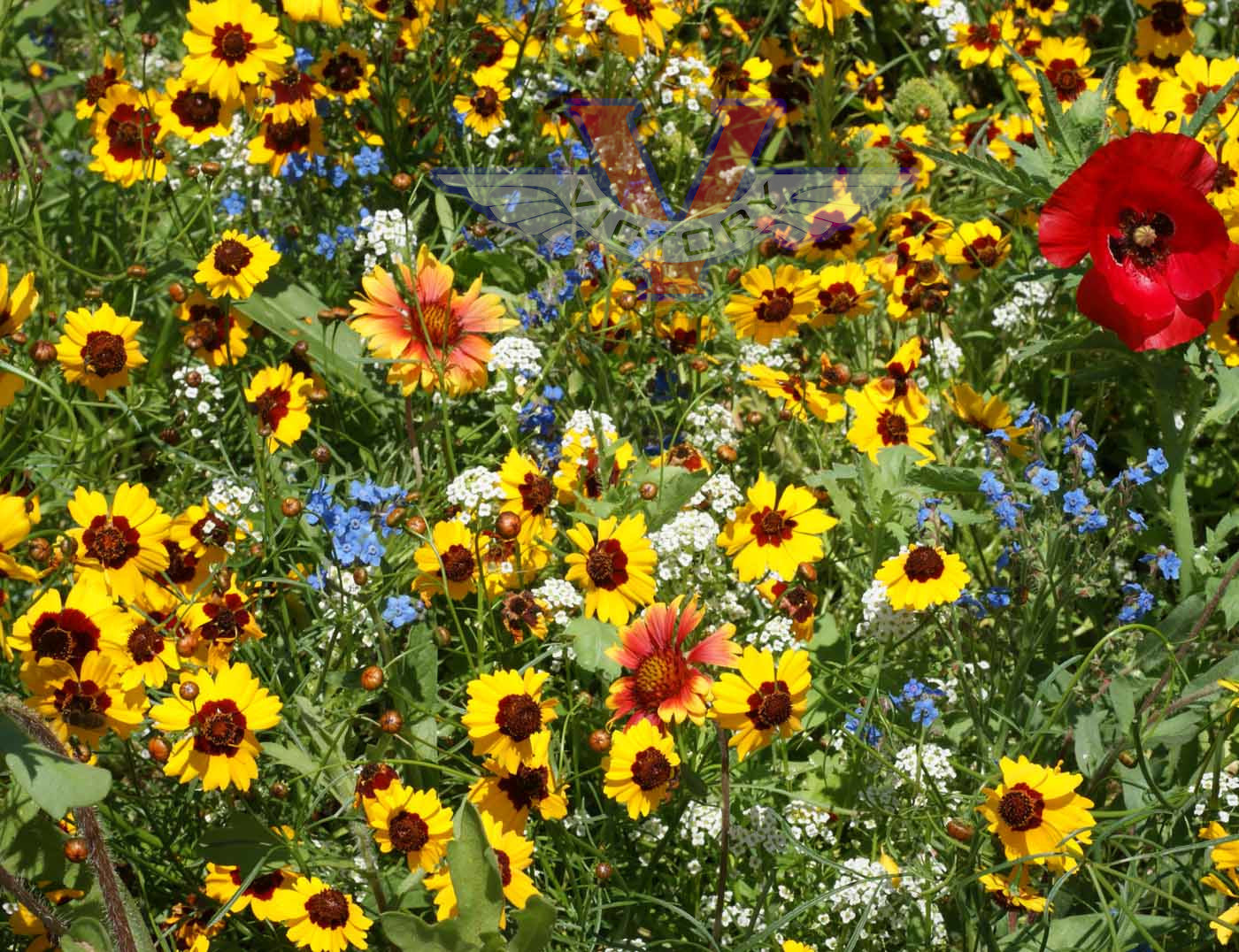The image is a detailed, photorealistic depiction of a garden teeming with wildflowers. The scene is richly populated with a variety of flowers and plants, showcasing a vibrant palette of colors. Dominating the garden are numerous flowers featuring yellow petals and brown centers. Interspersed among them are multi-colored flowers, particularly those with yellow and pink petals and a red center with a golden hue. Smaller clusters of delicate blue flowers and tiny white flowers add to the diversity, contrasting against the lush green of stems and grasses threaded throughout the garden.

Noteworthy is a striking large flower located towards the top right of the image. This unique bloom boasts vivid red petals with a black center encircled by a brown ring. The entire garden appears delightfully haphazard, creating a natural and untamed look. Additionally, the image contains a logo or watermark at the top center—a large red and blue "V" with a winged banner overlaying it. This banner has blue outlines and the word "victory" prominently displayed in black text. The overall scene is lively and intricate, drawing the eye to the myriad details of nature's splendor.